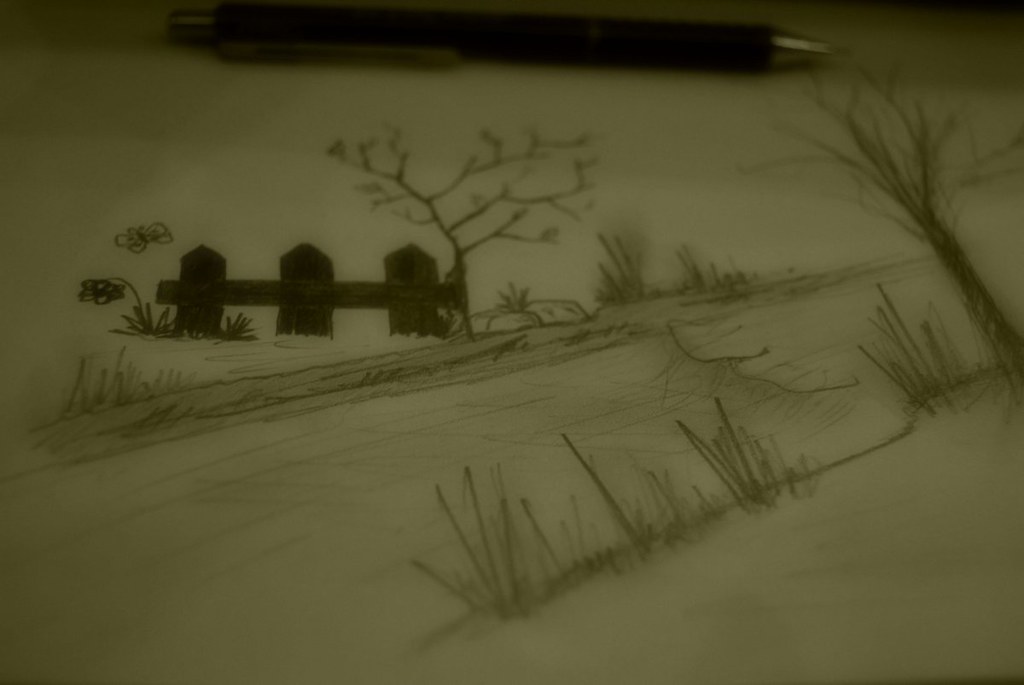This is a black and white pencil illustration on a white piece of paper, featuring a serene outdoor scene. At the top of the image, a black and silver pen, or possibly a mechanical pencil, rests horizontally, with its clip facing the camera. The central element of the drawing is a brown picket fence with three shaded pickets, running horizontally and partially obscured by a gently rippling creek that flows through the middle of the scene. Below the fence, a walkway is depicted, flanked by patches of grass and trees on either side. On the right side of the image, a hill rises gently, covered with long, wispy grass and a tree with bare branches. Another tree, also without leaves, stands next to the fence in the background. A butterfly flutters over the fence, while a slightly drooping flower can be seen near its left side. Scattered around are rocks and additional grassy areas, contributing to the tranquil, natural ambiance of the drawing. The image is wider than it is tall and contains no writing, people, or animals.